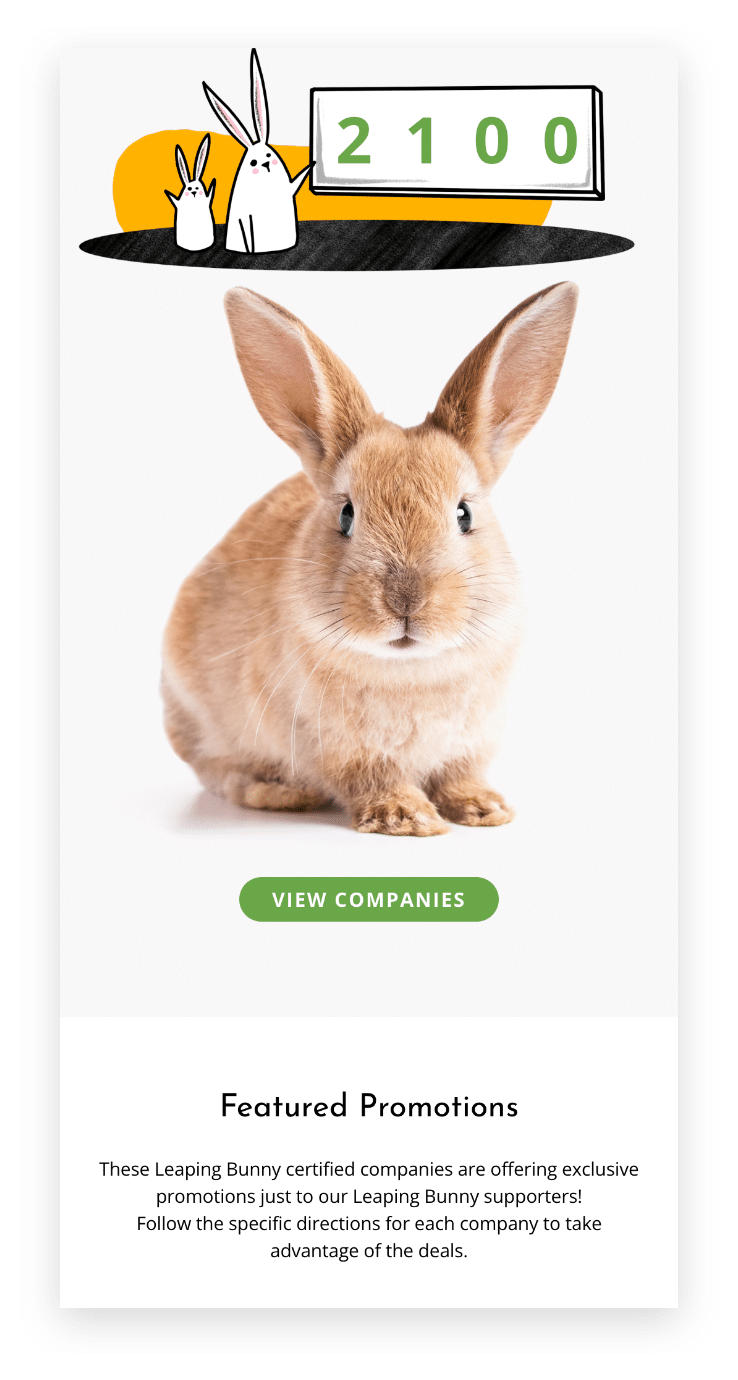The website displayed features a photograph of an adorable, real rabbit centered prominently on the page. The rabbit is tan-colored, with remarkably long, erect ears and a matching tan nose. It gazes directly at the camera, creating a captivating focal point. 

Below the image, there is a green bar with curved sides containing the text "View Companies." At the top of the page, there is an illustration of two bunny rabbits on a black plate, with one being noticeably larger than the other. Behind this illustration is a bubble-like image in orange, and the larger rabbit appears to be holding up a box labeled "2100."

At the bottom of the page, a section titled "Featured Promotions" describes that Leaping Bunny Certified Companies are offering exclusive promotions specifically for Leaping Bunny supporters. The text encourages viewers to follow specific directions provided by each company to make the most of these deals.

The website does not provide a specific company name or additional identifying information on this page, suggesting that it might be located a few pages deeper into the site.